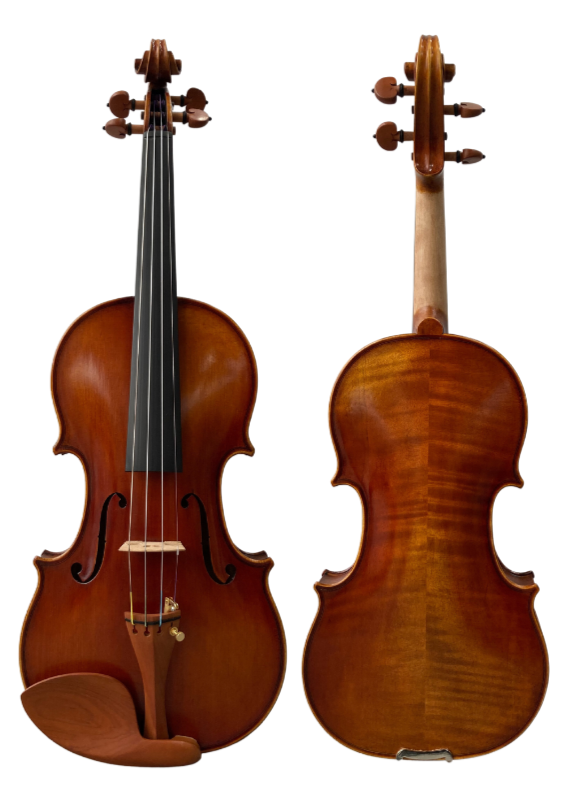In this detailed image, we have a presentation of two German violins showcasing different perspectives. The violin on the left side displays the front view, revealing its intricate design with four white strings stretched over a black neck and wooden chin rest. The one on the right side provides a view of the violin's back, featuring a white handle with tuning knobs on both sides at the top. Both violins are of the same height and exhibit a consistent wood grain finish in medium brown, although they possess a reddish-orange hue, adding to their vintage appearance. The violin on the right also has a noticeable metal clasp at the bottom and displays a subtle rainbow pattern in its wood grain. The background is a simple, uncluttered backdrop, ensuring full attention on the two meticulously crafted string instruments.